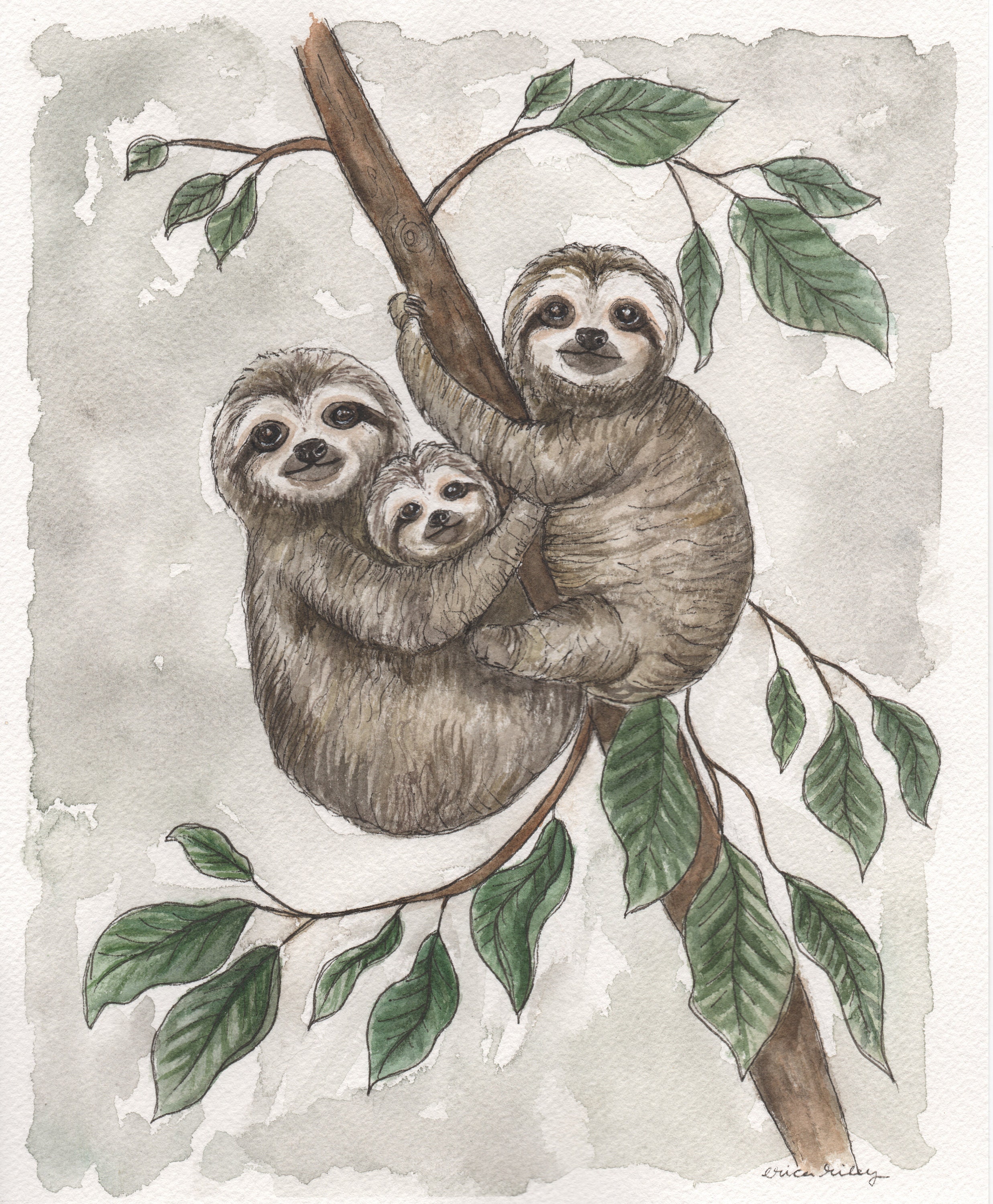This detailed pen and ink and watercolor art piece depicts a family of three sloths clinging to a tree branch. The main branch, with brown bark, extends from the top left to the bottom right of the image, sprouting additional smaller branches adorned with lush green leaves. Against a watercolor wash background of graded beige to dark gray, the sloths display distinctive features: grayish-brown fur, white faces, and black stripes extending from their eyes.

The largest sloth, positioned slightly left at the top of the branch, grips the branch with its left arm and leg while gazing directly outward. Below it, semi-upside down, a slightly smaller sloth mirrors this pose, also staring directly at the viewer. Nestled in the crook of this sloth's right arm, a tiny baby sloth peers out, adding an adorable touch to the scene. Together, these detailed elements form a harmonious and endearing portrayal of the sloth family amidst a serene, nature-inspired backdrop.